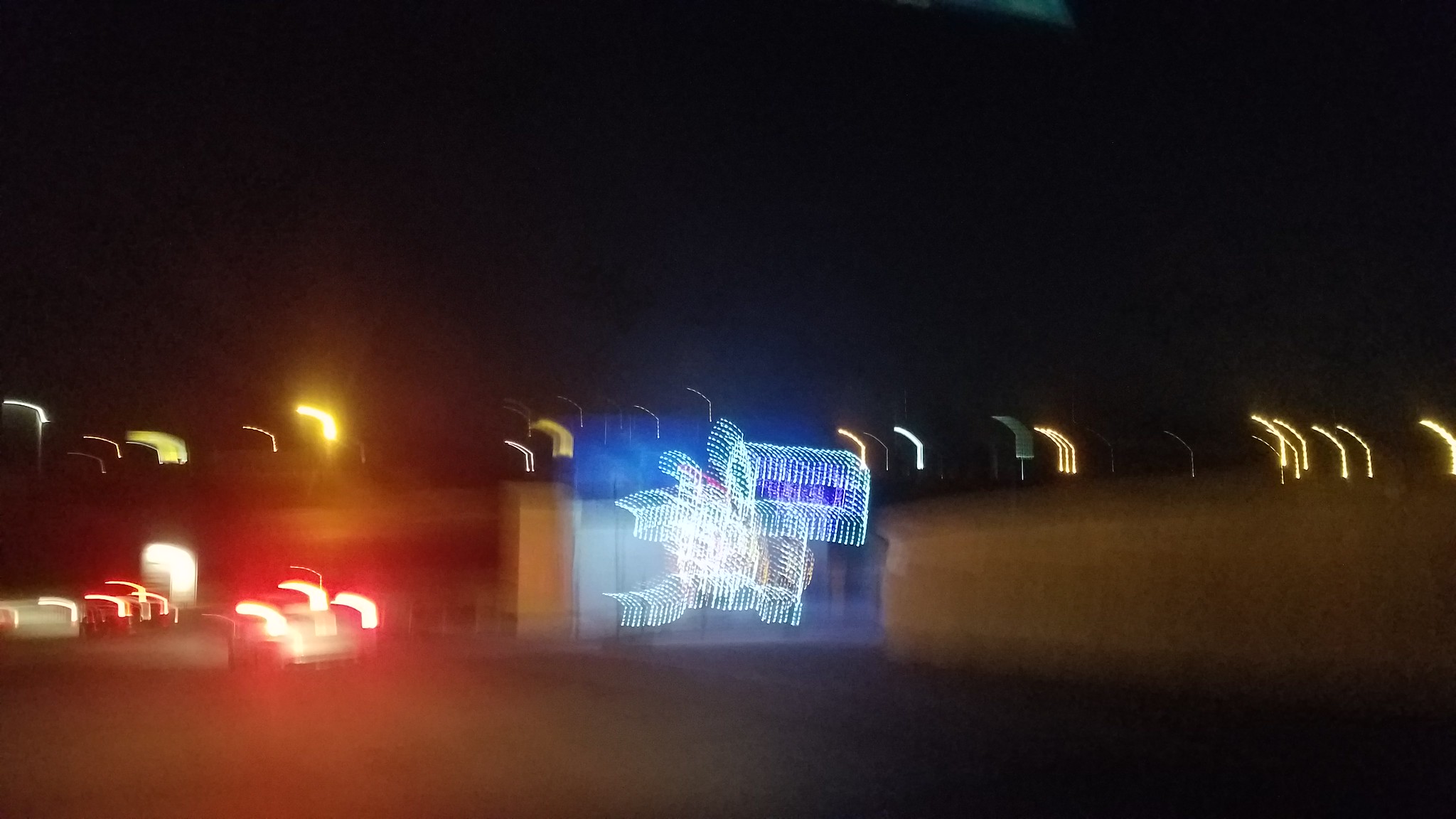This is a blurry, nighttime photograph exhibiting multiple image echoes, creating a jerky, doubled effect. The image is predominantly abstract, with a big black sky and rolling hills in the background. Numerous storage shed-shaped buildings are scattered across the landscape, some featuring roof lights that emit trailing, streaked echoes. There is also a vividly lit blue and white sign, adorned with a large bow, hinting at potential Christmas decorations or possibly signaling the entrance to a subdivision. In the bottom left, streaks of white and red lights are present, likely from the taillights of cars on a road that starts in the bottom right and slants diagonally left. Additionally, to the right, a streaky blue neon sign marks a potential turn, with a concrete barrier visible nearby. The entire scene is dotted with curved red, yellow, and white lights scattered throughout, contributing to the chaotic and abstract feel of the image.